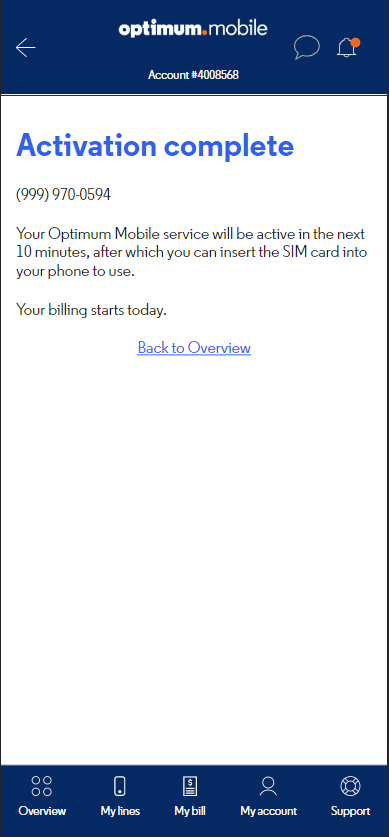This image is a detailed screenshot from a smartphone displaying a page with a clean white background and a sleek navy blue header and footer. At the top center of the header, the text "Optimum Mobile" is prominently displayed. The word "Optimum" appears in bold, white, lowercase letters followed by a small red dot and the word "Mobile" in lowercase white letters but not in bold. On the left side of the header is a white arrow pointing to the left, while the right side features a small chat bubble icon for live chat and a bell icon for notifications, with a red dot next to the bell indicating new notifications.

Beneath the header, in the center of the page, the text "Account" is displayed followed by the account number "4008568," also in white font. Below this section, against the white background, the text "Activation Complete" is prominently shown in large, bold, light blue letters. 

On the next line beneath "Activation Complete," a phone number "(999) 97050594" is displayed. Following this, in gray font, the message reads, "Your Optimum Mobile service will be active in the next 10 minutes, after which you can insert this SIM card into your phone to use." Below this, another message states, "Your billing starts today." Centered at the bottom of this section, a blue hyperlink text "Back to overview" is underlined, indicating a clickable link.

The footer, matching the navy blue of the header, includes five white icons and their corresponding labels from left to right: "Overview," "My Lines," "My Bill," "My Account," and "Support." Each label is accompanied by a relevant icon, making navigation intuitive and visually consistent.